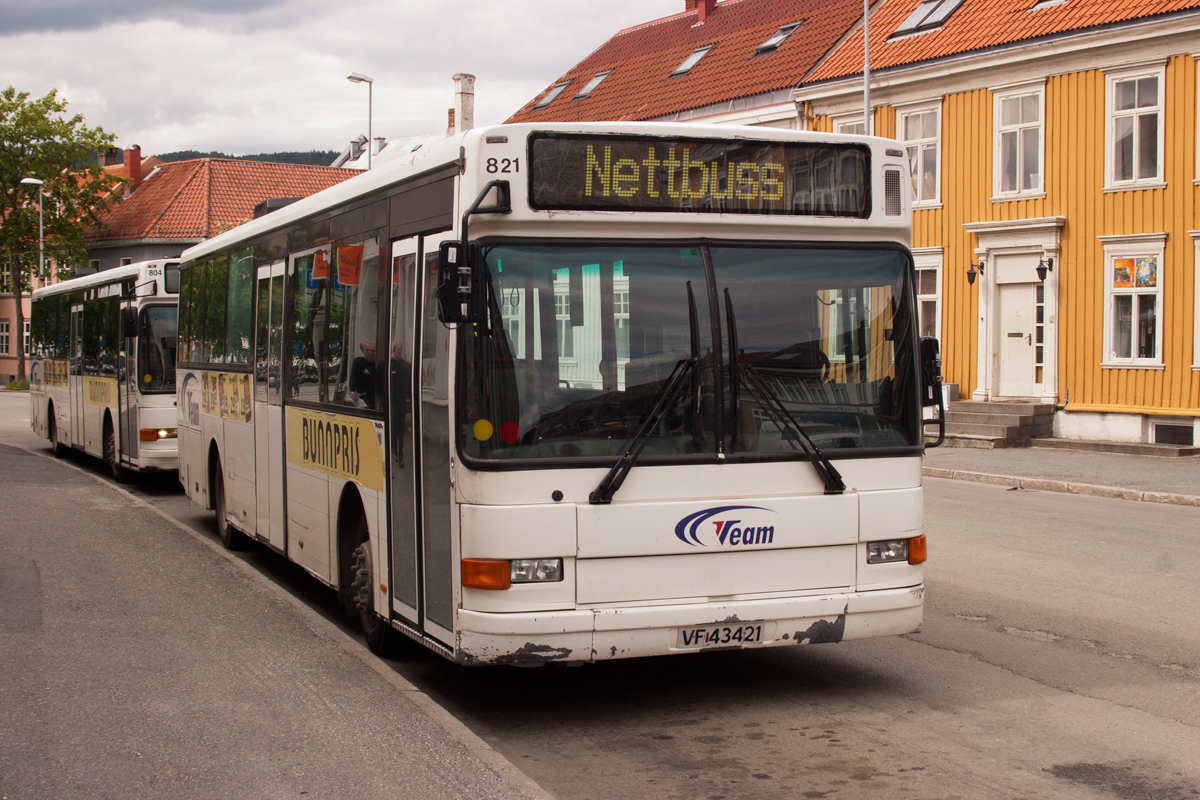This detailed photograph, taken on a gray, cloudy day in a town, captures an urban scene dominated by two large white public transportation buses parked along a clean, smooth street. The buses, both made by the VEAM company, have dark tinted windows along their sides and fronts. The leading bus prominently displays "NETBUS" as its destination and carries the number 821. Its license plate reads VF43421, with additional markings including the number VEAM. The second bus, similarly colored, is parked directly behind the first.

In the background, partially obscured by the buses, stand two buildings with distinct red terracotta roofs. The building to the left features a chimney and a narrow tree with a brown trunk and green leaves beside it. To the right, partially visible, is a yellow building with white-framed windows and a door. There is a touch of an orange-tiled house further in the backdrop. The vertical slat faces of the buildings add a textural element to the scene, and skylights are visible on the roofs. The sky above is mostly covered by large white clouds, with hints of grayish-blue peeking through, contributing to the overcast ambiance. No people are seen in the photograph, and the doors of the buses remain closed, suggesting a quiet moment in this urban setting.